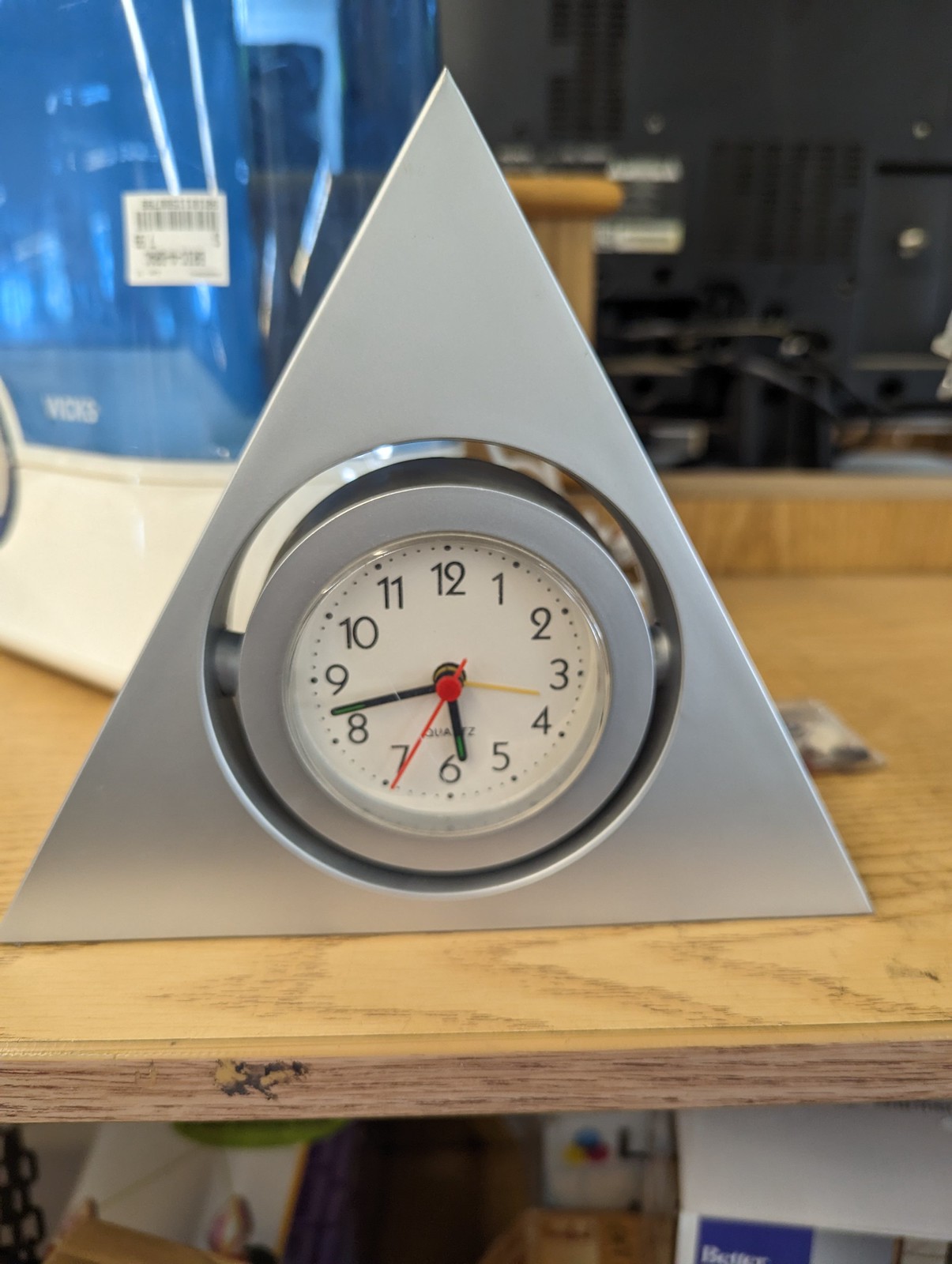The image is a color photograph depicting a modern, silver triangular clock centrally positioned on a light wooden table. The triangle's two longer sides frame a circular clock face in the middle, which has a white background adorned with large black numbers and smaller black dots marking the minutes. The clock features black hour and minute hands, along with a red second hand pointing at the seven, indicating a time of approximately 5:42. The clock is encased in a silver ring and gray border, adding to its sleek, modern design. Surrounding the scene, the wooden table extends horizontally with noticeable light brown grain patterns and includes a slight ledge at the back. Situated behind the clock to the left, a blue water pitcher with a white base is visible. The background comprises a blurred office or studio setting and a black wall, with some indistinct items and white boxes scattered beneath the table.